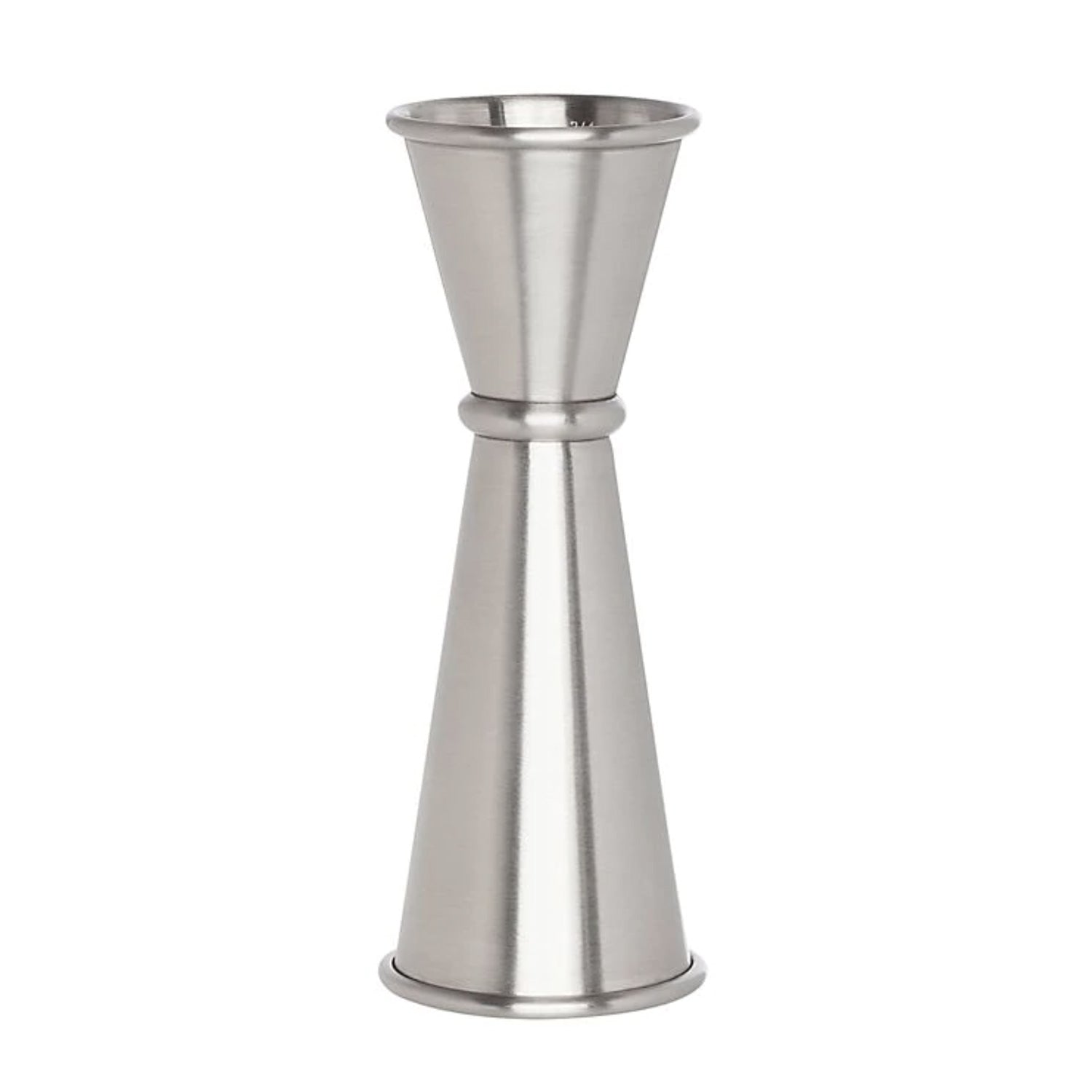The image is a detailed photograph of a unique metallic object placed against a white background. The object appears to be a sophisticated steel container or holder, composed of two conical sections that are seamlessly merged. The bottom two-thirds of the structure is a larger, upright cone, while the top one-third is a smaller, inverted cone, creating an hourglass-like shape. The point where these cones meet is reinforced by a thick, shiny metal band that encircles the entire object. This band is distinct and possibly white-lined, providing a contrasting aesthetic. The surface of the object is highly polished and reflective, suggesting a well-crafted, stainless steel material. The design features a smaller opening at the bottom and a broader opening at the top. Despite its elegant and functional appearance, the exact purpose of this container remains unidentified, though it could plausibly serve as a stylish egg holder or possibly a decorative piece.